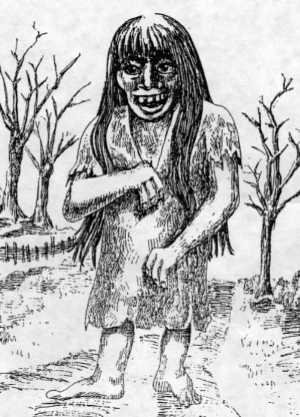This is a vertically oriented, black and white pencil-illustrated drawing on white or light beige paper, resembling the style of "Where the Wild Things Are." The central figure, standing in a barren landscape, is a disturbing blend of adult and child features: a distorted adult face with pronounced dark shadows, crooked teeth, and a very large nose, framed by long black hair with bangs extending down to the waist. The body, child-sized and disproportionate, with noticeably short arms and legs, is clad in a ragged white dress-like garment. The figure has only three fingers on each hand and fewer than five toes on each foot. The scene is set against a forest or field backdrop featuring three leafless trees and a small fence made of broken tree limbs. Grass and small plants can be seen near the feet, suggesting a rural or farmland area. The eerie character is positioned prominently in the center of the composition, contributing to the surreal, unsettling atmosphere.